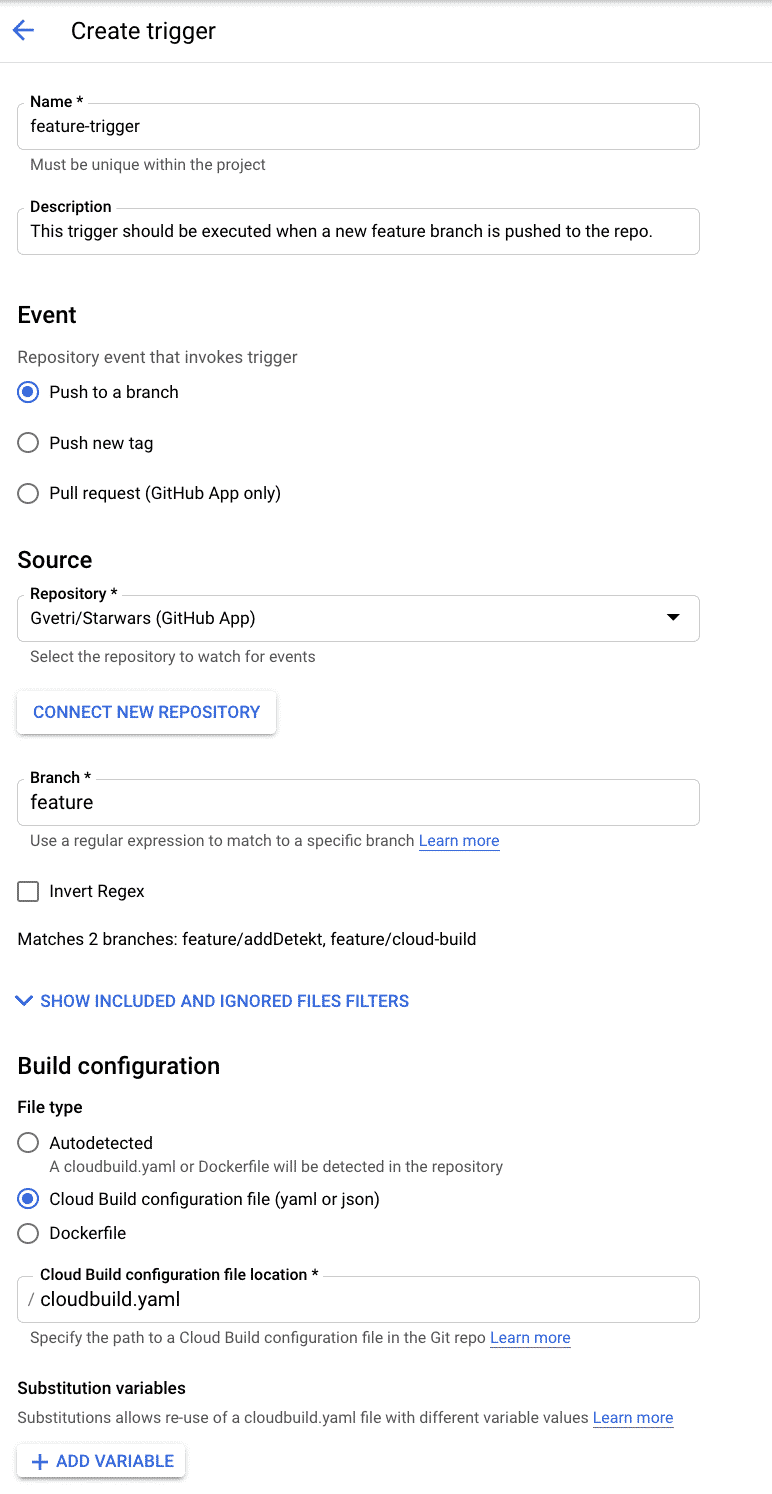**Screenshot: Setup for a Feature Branch Trigger in a Repository**

The screenshot illustrates the detailed steps involved in setting up a feature branch trigger within a repository. 

1. **Trigger Creation:**
   - **Title**: "Create Trigger"
   - **Name Field**: "Feature Trigger"
   - **Description**: "This trigger should be executed when a new feature branch is pushed to the repository."

2. **Event Selection:**
   - **Event**: "Repository event that invokes trigger"
   - **Options Available**:
     - "Push to a branch" (selected)
     - "Push new tag"
     - "Pull request (GitHub App only)"

3. **Source Configuration:**
   - **Repository**: 
     - "Repository: 'givetry/starwars'"
     - **Connect New Repository Button**: Located below the repository selection.
   - **Branch**:
     - Branch name: "feature"
   - **Invert Match**:
     - An empty checkbox labeled "Invert Match"
   - **Matching Branches**:
     - "feature/add-detect"
     - "feature/cloud-build"

4. **File Filters and Build Configuration:**
   - **File Filters**:
     - An option to "Show included and ignored files filters"
   - **Build Configuration**:
     - **File Type**: "Auto-detected"
     - **Cloud Build Configuration File**:
       - "YAML or JSON" (selected)
       - Other options: "Dockerfile"
     - **Configuration File Location**:
       - "/cloudbuild.yaml"

5. **Substitution Variables:**
   - Section for "Substitution Variables"
   - A button labeled "Add Variable"

This setup screen is designed to configure an automated trigger that activates specific build actions when changes are pushed to designated feature branches in the repository.